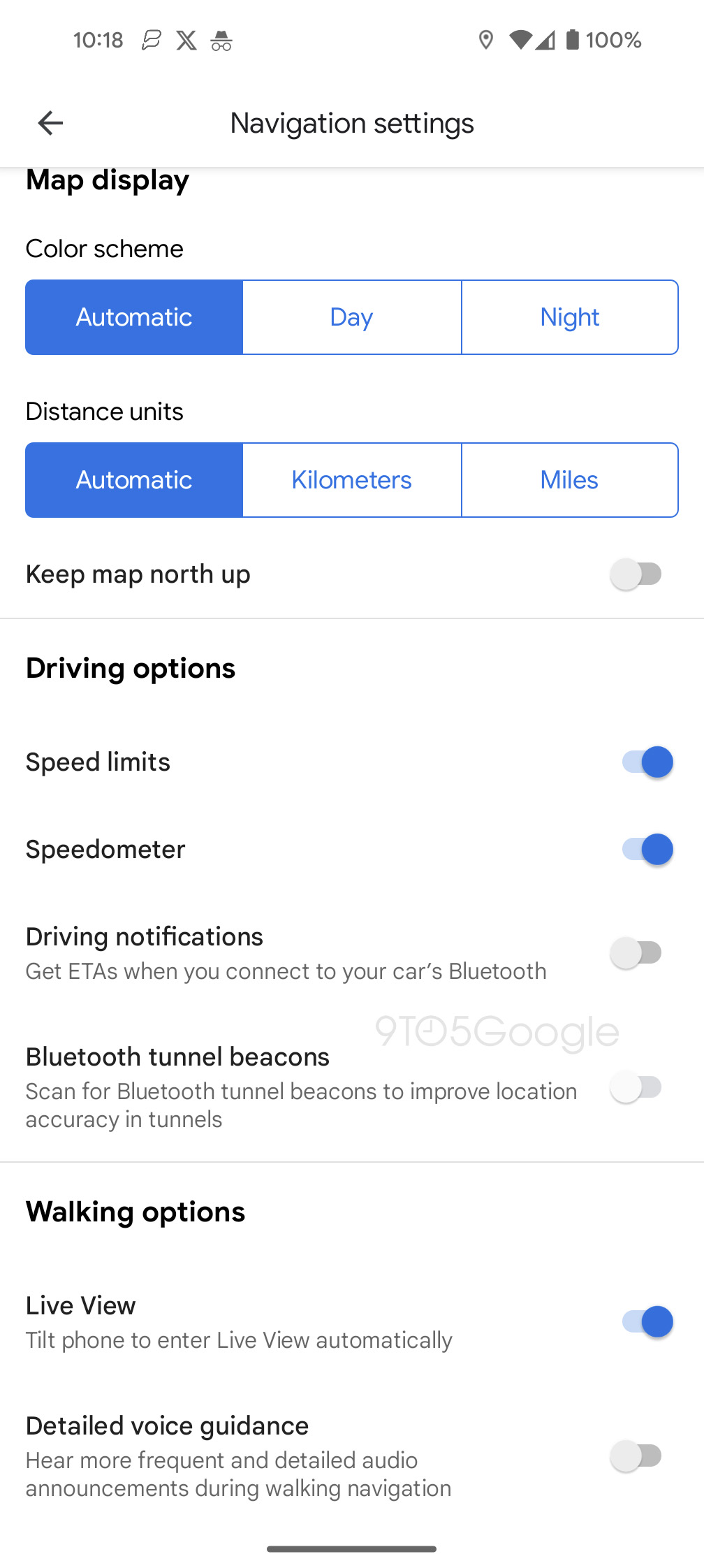The image is a screenshot from a mobile phone displaying the settings page of a navigation application. The background is white with black text. In the upper left corner, the time is indicated as 10:18, while various mobile icons such as Wi-Fi, 100% battery, and signal strength are displayed on the right.

At the top centre of the screen, there is a navigation bar with a back arrow for returning to the previous menu. Below this, the settings options begin with "Map Display," which includes "Colour Scheme." There are three rectangular selections for this setting: "Automatic" (selected and highlighted in blue), "Day," and "Night," both of which are in blue text and situated on the right.

The next section is "Distance Units," with "Automatic" selected and highlighted in blue on the left. Other options, "Kilometres" and "Miles," are listed on the right in white text with blue descriptions.

Below this, there is a setting option to "Keep Map North Up," which has an unselected slider button. Following this section is "Driving Options," with several toggles: "Speed Limits" (slider turned on and highlighted in blue), "Speedometer" (selected and on), and "Driving Notifications" (option to get ETAs when connected to the car’s Bluetooth, which is off).

There appears to be a grey watermark near these settings, possibly reading "Google" or "9105 Google," though it is difficult to discern clearly. Another setting called "Bluetooth Tunnel Beacons," described as scanning for Bluetooth tunnel beacons to improve location accuracy, is also turned off.

"Walking Options" are listed next, with "Live View" set to on, allowing the phone to enter live view automatically when tilted. "Detailed Voice Guidance," which provides more frequent and detailed audio announcements during walking navigation, is turned off.

At the bottom of the screen, there is a small, thin horizontal line that extends about a third of the way across the page, centered.